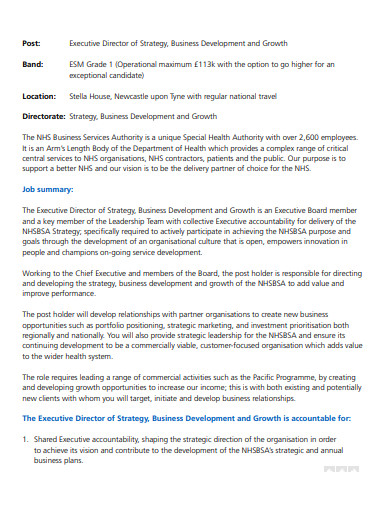The image showcases a detailed job posting for the position of Executive Director of Strategy, Business Development, and Growth. This role is classified under Band ESM Grade 1 with an operational maximum salary of £113,000, with potential for a higher salary for an exceptional candidate. The position is based at Stella House in Newcastle-upon-Tyne and requires regular national travel.

The posting identifies that the job falls within the Directorate of Strategy, Business Development, and Growth. The NHS Business Services Authority (NHSBSA), a unique special health authority with over 2,600 employees, operates as an arm's length body of the Department of Health. It provides a broad range of essential central services to NHS organizations, NHS contractors, patients, and the general public. The NHSBSA's mission is to support a better NHS and its vision is to become the delivery partner of choice for the NHS.

The job summary emphasizes the need for critical skills, highlighting that the Executive Director will have shared executive accountability for guiding the strategic direction of the organization. The role involves significant responsibility for shaping and contributing to the development of the NHSBSA's strategic and annual business plans.